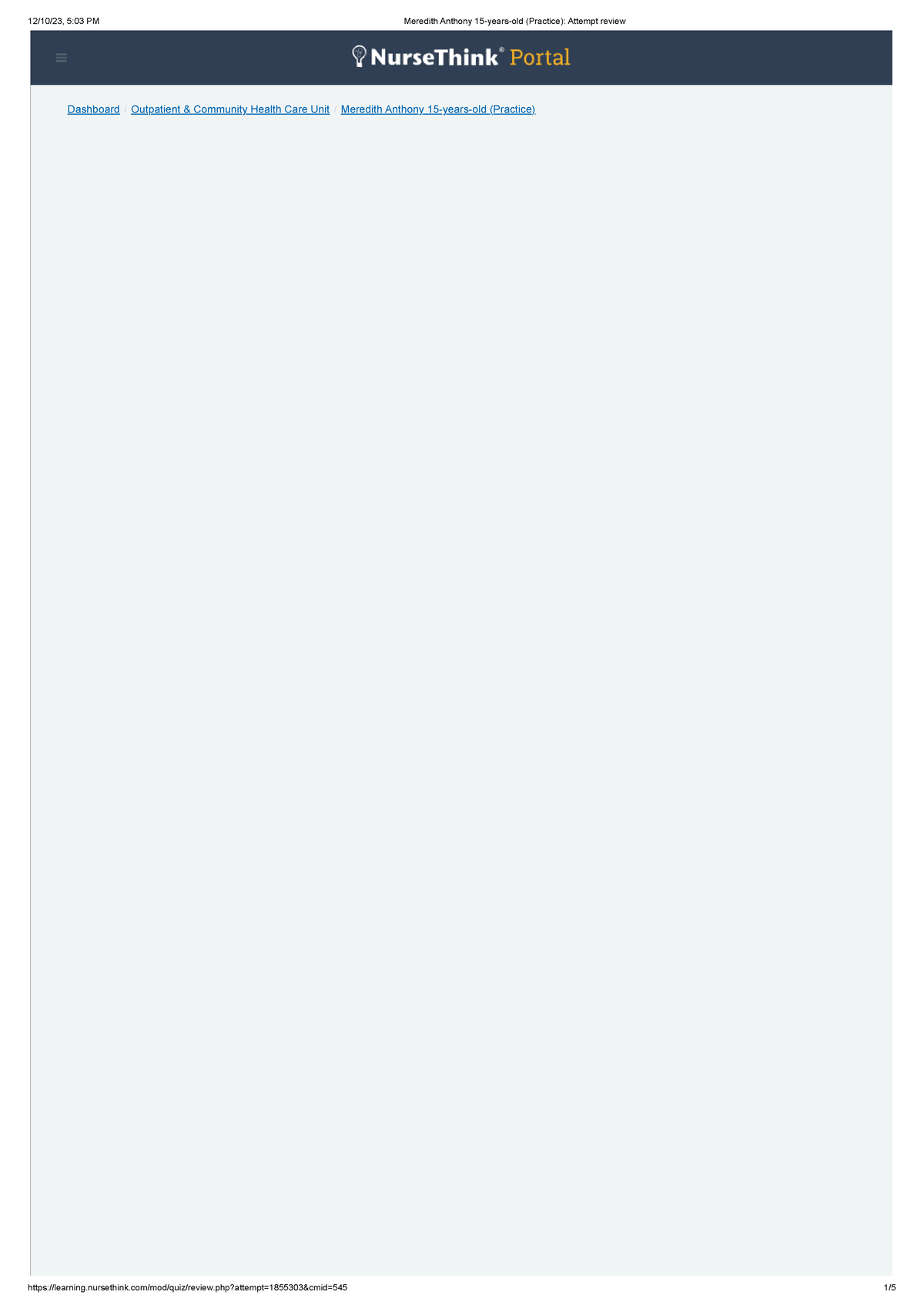This image appears to be a screenshot of a website interface. At the top of the image, there is a timestamp: "12/10/23, 5:03 PM." Centered beneath this, the text "Meredith Anthony, 15 years old (Practice)" is prominently displayed, followed by the phrase "Attempt Review."

A dark gray banner stretches across the width of the image beneath this text. In the center of the banner, the words "NurseThink" are displayed in white font alongside a light bulb icon. The word "Portal" appears next to it in yellow font.

Below the banner is a large, mostly empty space with a light gray background. At the top of this section, several links are visible in blue, underlined text: "Dashboard," "Outpatient," and "Community Health Care Unit."

The name "Meredith Anthony, 15 years old (Practice)" appears again just below these links. The rest of the space below is largely vacant. In the bottom right corner of the image, there is a URL for the practice attempt and the text "1/5."